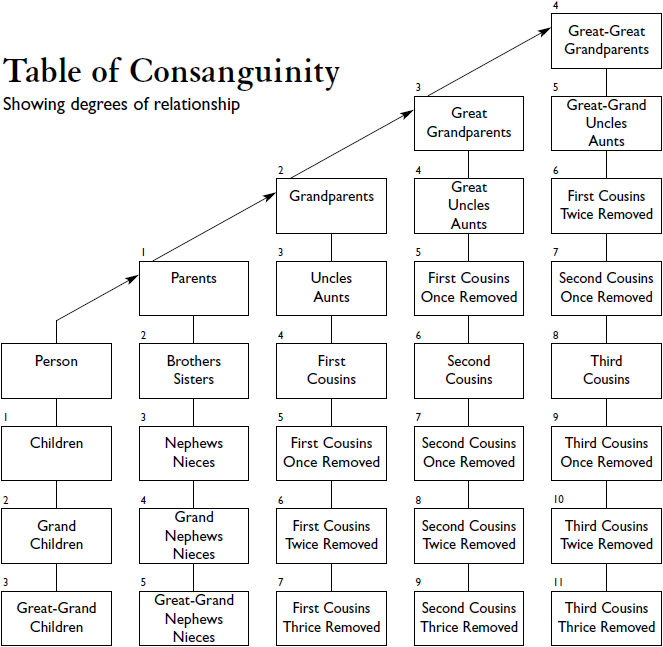The screenshot showcases a detailed table of consanguinity, illustrating the degrees of familial relationships across multiple columns. The chart expands horizontally, with each subsequent column containing an increasing number of rectangles, starting with four in the first column and incrementally adding one more rectangle per column until there are eight rectangles in the final column.

In the first column, the entries include "Person," "Children," "Grandchildren," and "Great-Grandchildren." The second column expands to include "Parents," "Brothers," "Sisters," "Nephews," "Nieces," "Grandnephews," and "Great-Grandnieces." The third column further adds "Grandparents," "Uncles," "Aunts," "First Cousins," "First Cousins Once Removed," "First Cousins Twice Removed," and "First Cousins Thrice Removed."

The fourth column lists "Great-Grandparents," "Great-Uncles," "Great-Aunts," "First Cousins Once Removed," "Second Cousins," "Second Cousins Once Removed," "Second Cousins Twice Removed," and "Second Cousins Thrice Removed." Finally, the fifth column details "Great-Great-Grandparents," "Great-Granduncles," "Great-Grandaunts," "First Cousins Thrice Removed," "Second Cousins Once Removed," "Third Cousins," "Third Cousins Once Removed," "Third Cousins Twice Removed," and "Third Cousins Thrice Removed."

This visually structured table provides a comprehensive reference for understanding the degrees of kinship within an extended family tree.